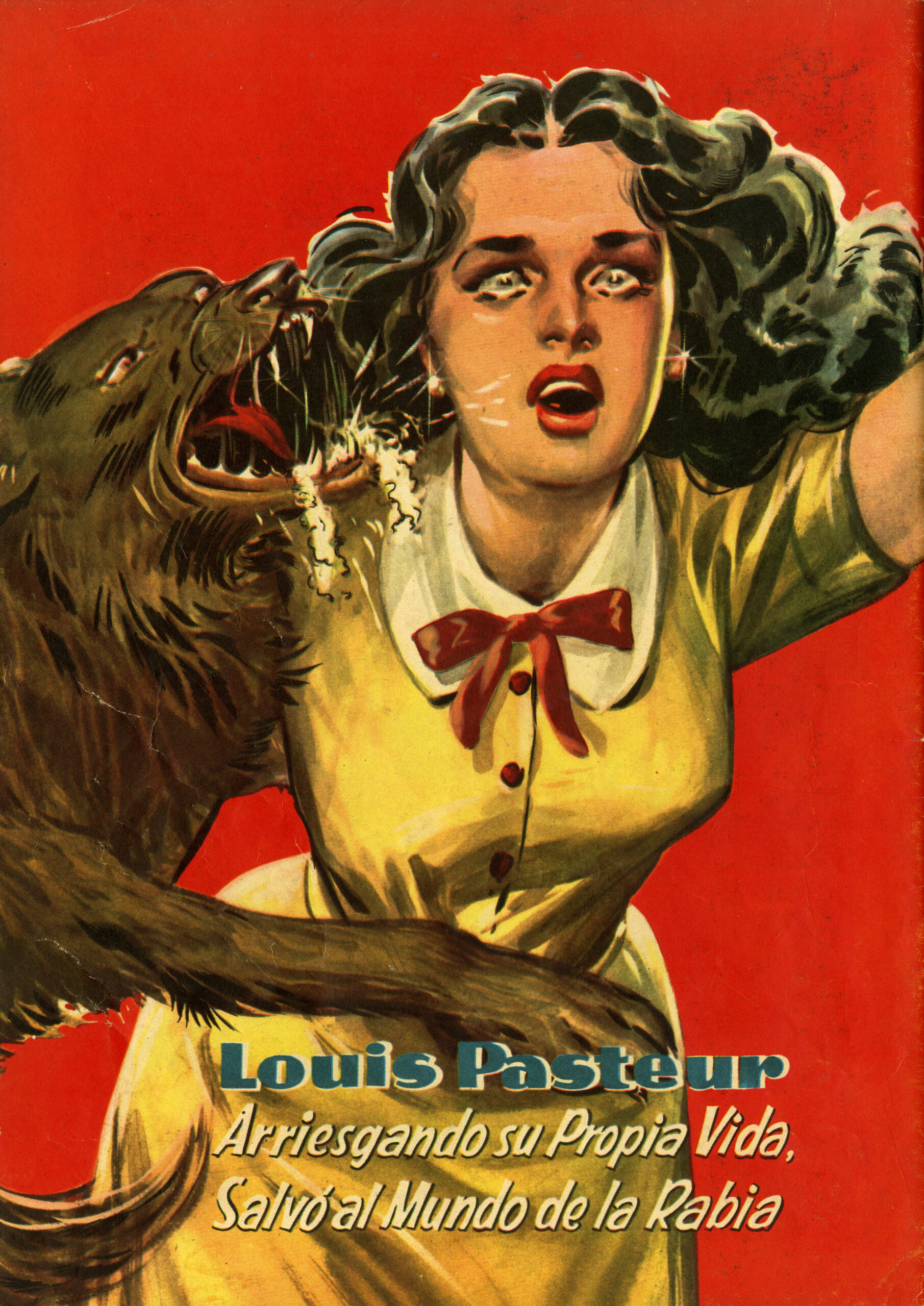In the image, a terrified woman with curly black hair, red lipstick, and diamond stud earrings gazes towards the viewer, her eyes wide with fear and tears streaming down her face. She is dressed in a yellow dress adorned with red buttons, a white collar, and a red bow. Her right arm reaches out but is cut off in the image, revealing only a bit of skin from her short sleeve. The background is a vivid red. To her left, a menacing werewolf with brown and gray fur, a foaming mouth, and a red tongue lunges at the diamond stud earring on her left ear. The werewolf's eyes and nose are defined with brown beads. Over her body, text reads, "Luis Pastor," and additional Spanish text states, "Con su propia vida ha salvado al mundo de la rabia," indicating that Luis Pastor has dedicated his life to combating rabies.